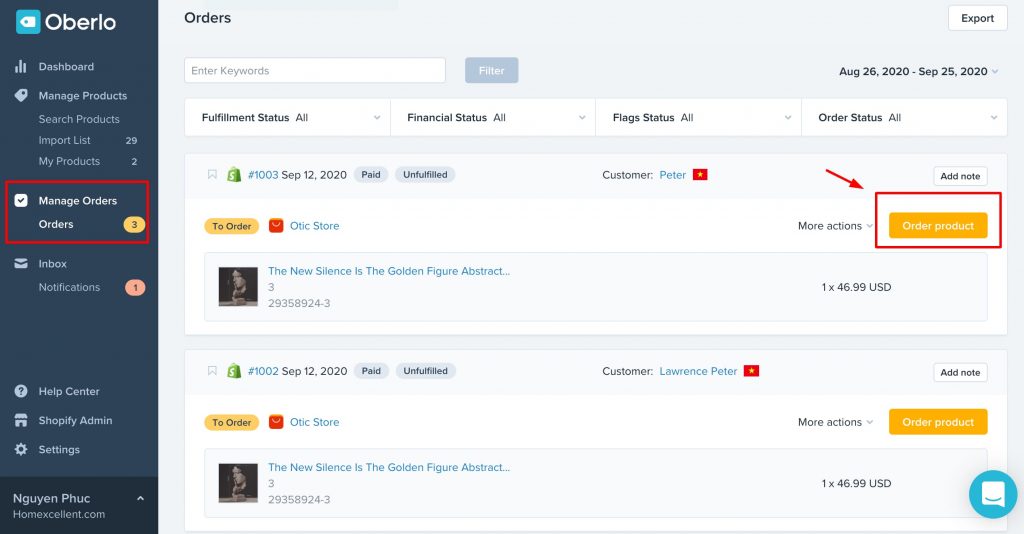Here’s a revised and detailed caption for the image described:

---

The webpage features a streamlined interface characterized by its distinct color schemes. In the upper left-hand corner, a sky blue icon is prominently displayed beside the site name "Arborello," set against a dark blue background. Below this header, a sidebar menu lists several key sections: "Dashboard" with a graph icon, "Manage Products," "Search Products," and "Port List" marked by the number 29, and "My Products" indicating the number two. 

A red-highlighted box with checked borders showcases "Manage Orders" and "Orders," accompanied by a yellow-highlighted number three. Further down, an envelope icon precedes "Inbox," followed by "Notifications" with a circled number one. The menu continues with "Help Center," "Shopify Admin Settings," and "Nugent Book," concluding with "Homeexcellent.com" in a black box with an upward-pointing arrow.

In the page's central area, the header "Orders" is prominently displayed above a keyword entry section and a filter button. Towards the upper right, an "Export" button is visible. Two order information sections are presented, each featuring the same media image and labeled "Silence is Golden Figure Abstract." The first order product is highlighted within a red-bordered box, while the second is not.